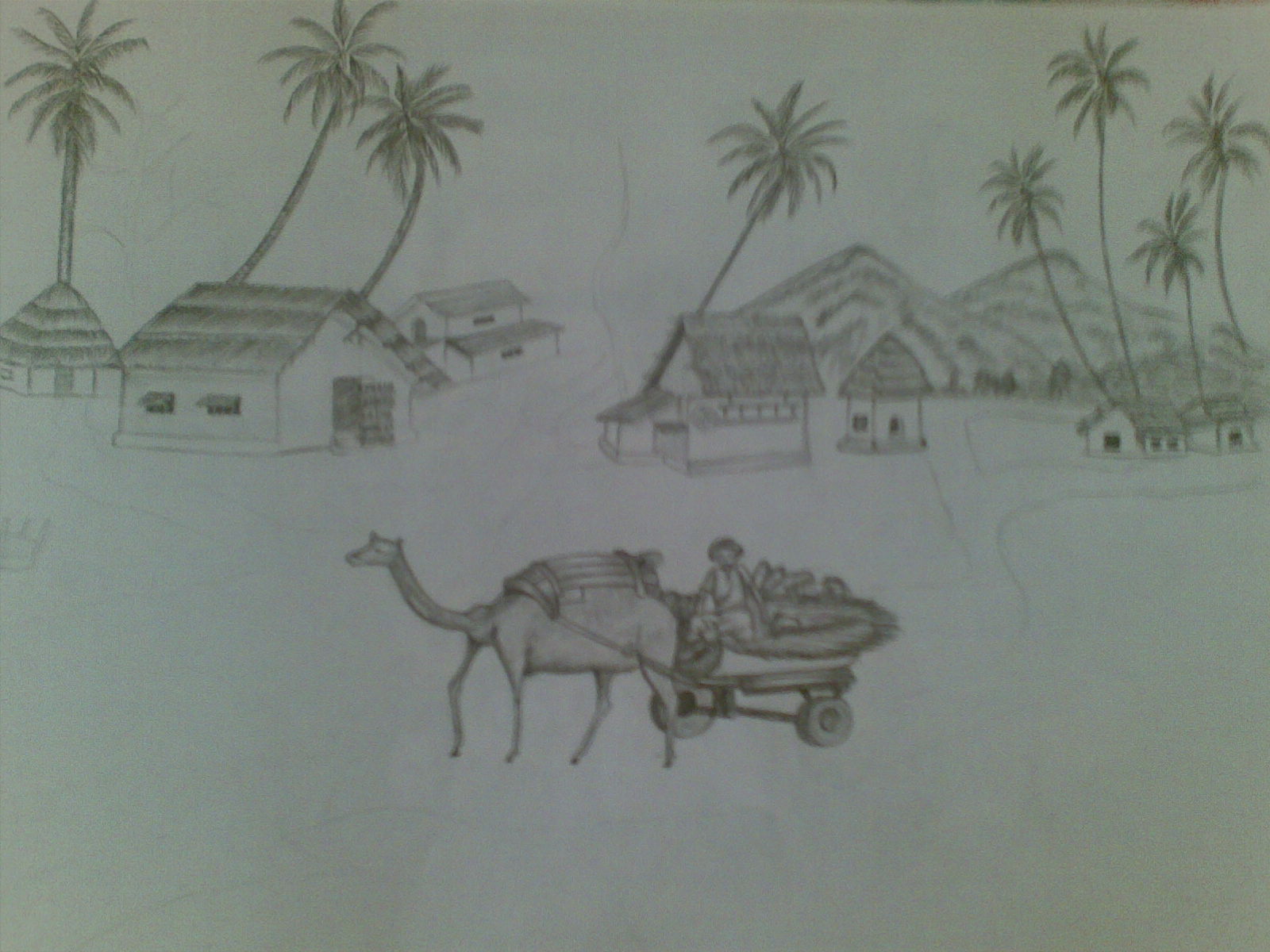This detailed pencil drawing, created by a novice or young artist, captures a rustic scene rendered on white paper that appears dark grey under indoor lighting. Central to the composition and occupying the bottom half of the page is a camel, oriented towards the left, pulling a two-wheeled cart. Seated on the cart is a man accompanied by assorted products. Behind the cart, a road trails off into the distance. The upper portion of the artwork features an array of houses with thatched roofs, interspersed with multiple palm trees. In the background to the right, two tall hills rise into view, adding depth to this picturesque and charming depiction of a quaint, rural landscape.